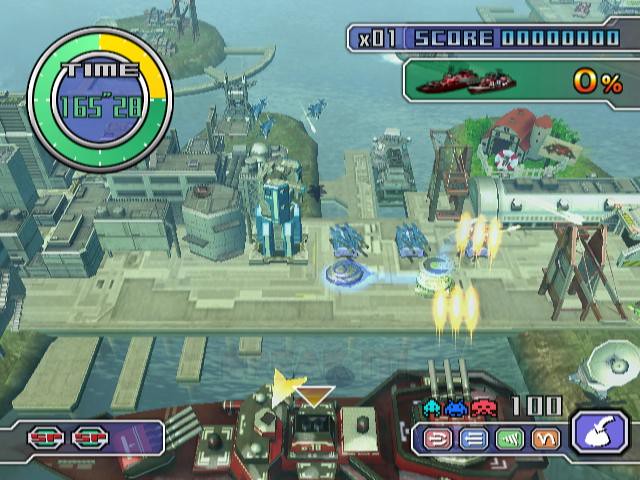This image is a detailed screen capture from a high-tech video game, showcasing a vibrant 3D scene of a high-tech cityscape situated on a bridge or peninsula surrounded by water. In the foreground, there is a prominent red battleship equipped with three turret guns, actively firing. The ship's guns appear to be directing their fire at a small, farm-like building with a silo, located on the right side of the image. The blasts from the guns are visibly arcing toward this target. The cityscape features tall, futuristic buildings and additional structures that resemble a dock or pier, with other vessels possibly visible in the scene.

The gaming interface is also prominent: on the left side of the screen, a time icon indicates the remaining time for the current level or quest; on the right side, the player's score, the number of lives left, a zero percentage, and additional in-game statistics are displayed. The bottom corners of the screen have various panels, likely showing inventory, powers, and other game settings. Alien-like pixel art, reminiscent of classic games like Space Invaders, adds a layer of detail to the foreground. Helicopters are seen flying overhead, and enemy tank-like vehicles are positioned on the roads, against which the player appears to be fighting. The overall scene suggests intense gameplay as the player maneuvers the battleship to combat enemy forces and defend or attack key structures in the city.